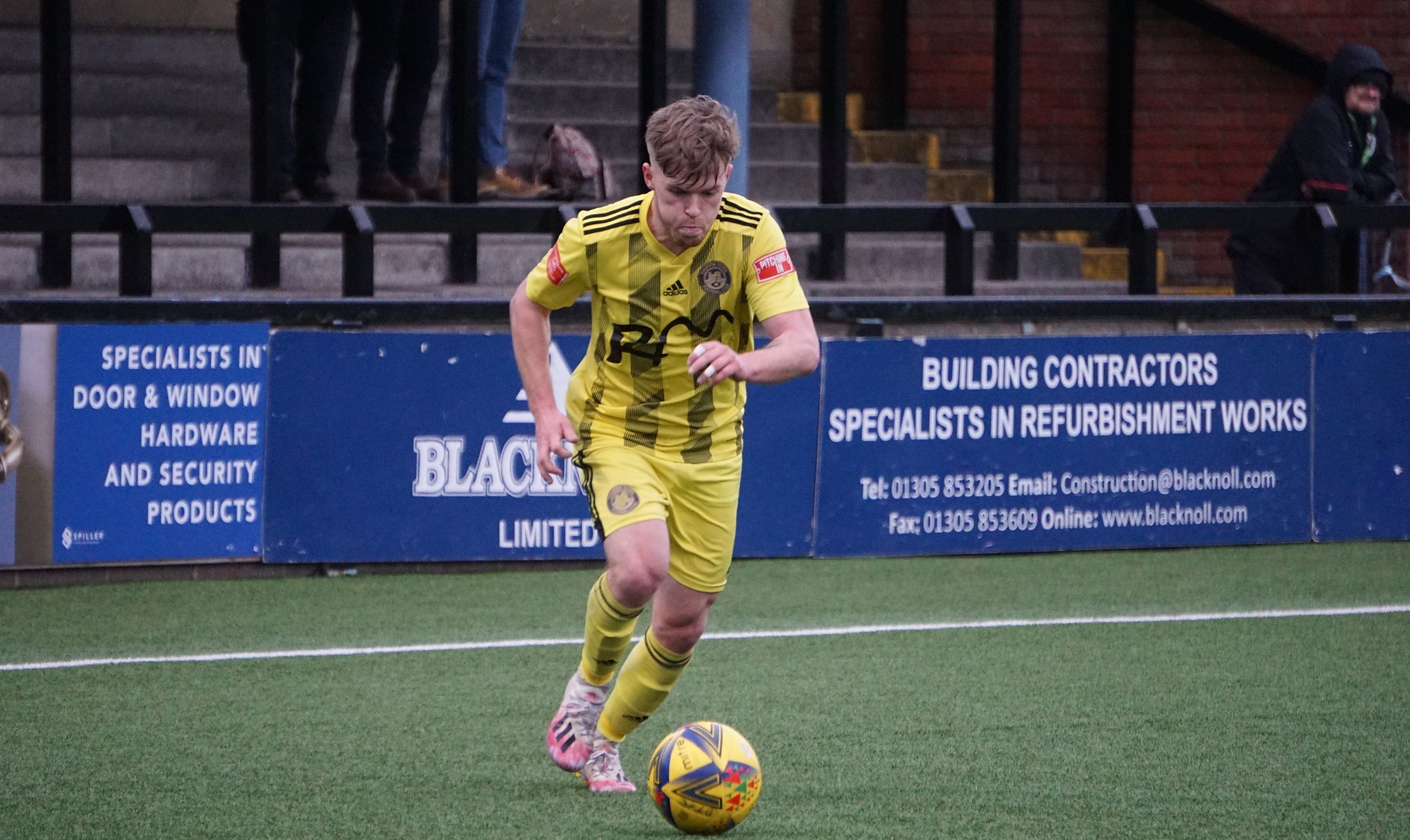The photograph captures an intense moment during a soccer match. Central to the image is a focused soccer player wearing a bright yellow jersey emblazoned with "RM". He pairs this with yellow shorts, long yellow knee-high socks, and white shoes splashed with pink paint. The player, a white man with short brown hair and shaved sides, is intently looking down at a vibrant yellow soccer ball, adorned with various colors and blue arrows, with a look of concentration and a slight frown as if puffing out air. 

In the background, the scene displays sparse attendance in the bleachers with only three visible spectators and another person seated at the top right corner. The left side of the background has concrete steps edged in yellow, where the lower part of some jeans-clad legs are visible. Near the brick wall on the right, a person in a black hooded jacket leans on a railing. The soccer field itself is bordered by blue signage promoting a building contractor, featuring white lettering that reads: "Building Contractors, Specialists in Refurbishment Works. TEL: 01305-853205, Email: construction@blackknoll.com, Fax: 01305-853609, www.blackknoll.com," and on the left, it mentions "Specialist in door and window hardware and security products". The lush green turf contrasts with the vibrant attire of the player, bringing the entire scene to life.